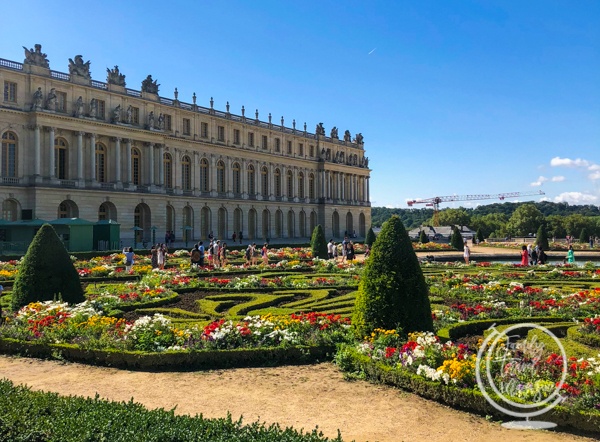The image depicts an elegant, sprawling French-style palace set against a clear blue sky with a few white, puffy clouds. The grand structure, possibly a former court or university building, spans three to four stories and is constructed from brown sandstone with tall, large windows and ornate stone columns and sculptures adorning the roof. The palace's majestic facade is complemented by a meticulously maintained, vibrant garden that stretches across the foreground. This garden features finely cut green shrubs and an assortment of colorful flowers, including whites, reds, and yellows, intricately woven along the edges of a central maze. The maze, flanked by dirt pathways, guides visitors who are scattered throughout, some pausing to take pictures of the breathtaking architectural beauty. In the distant background, an industrial crane hints at ongoing construction work, adding a modern touch to the classical scene.